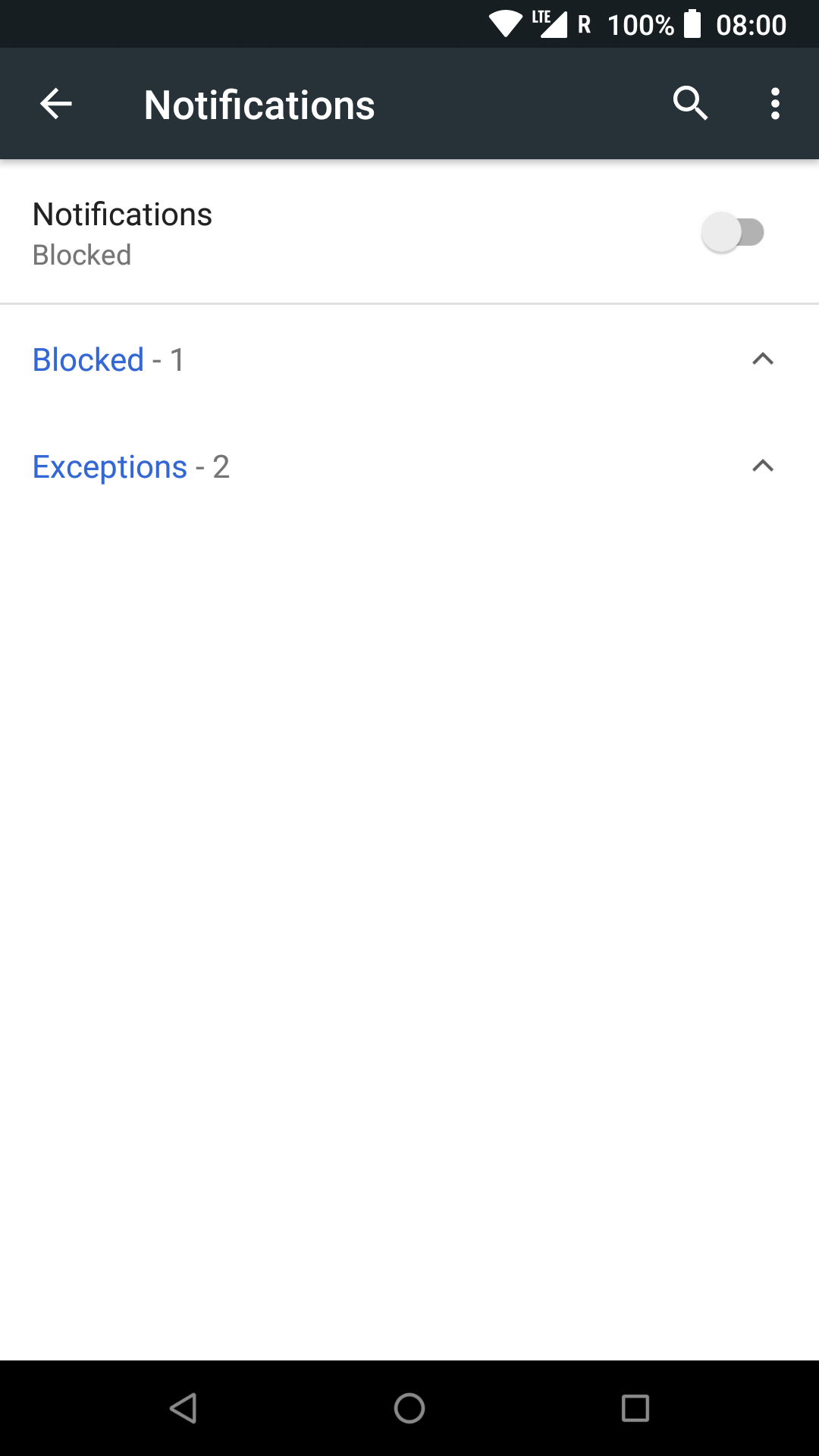The image depicts a notification settings screen on a smartphone. At the top right corner, the status icons include a fully connected Wi-Fi symbol, a cellular connection icon accompanied by an 'R,' indicating roaming, and a battery life indicator showing 100%. The current time is clearly displayed as 08:00.

Directly below this, the header section features the word "Notifications" in white text on a very dark gray background. Adjacent to it, there is a search icon and a vertical ellipsis (three dots) in white.

Underneath the header, the screen states "Notifications blocked," followed by the labels "Blocked," with the number "1" next to it, and "Exceptions," with the number "2" beside it. The text "Blocked" and "Exceptions" are highlighted in blue, whereas the numbers are in gray. 

The main background of this section is predominantly white. Two upward-pointing arrows are located to the right of the labels, pointing towards the right side of the screen.

At the very bottom, there's a horizontal rectangular black bar. This bar contains three navigation icons in gray: an arrow pointing to the left on the left side, a circle in the center, and a square on the right side.